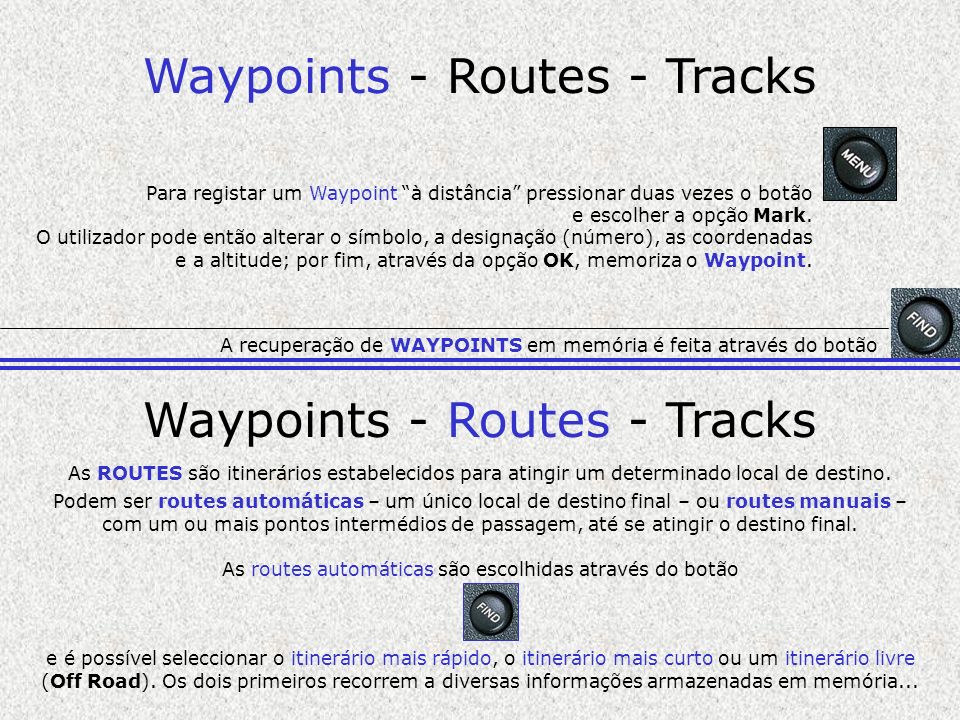The slide presentation titled "Waypoints, Routes, and Tracks" features comprehensive text in Portuguese, explaining the concepts of waypoints, routes, and tracks. The slide is organized into two distinct sections: the top section highlighted in purple focuses on waypoints, while the lower section features routes. The overall background is gray speckled with white texture, creating a subtle yet textured appearance.

The top section is dedicated to waypoints and is marked by blue text, distinguishing it from the black text used for routes and tracks. The corresponding Portuguese text elaborates on the functionality of a waypoint. Additionally, three graphics on the right side of this section display buttons labeled "Menu" and "Find."

The lower section centers on routes and is divided from the upper part by two thin blue lines. Similar to the top section, this one also includes Portuguese text and another "Find" button graphic, this time positioned in the lower center. Black squares containing white lettering are scattered throughout the slide, providing further visual elements to the presentation.